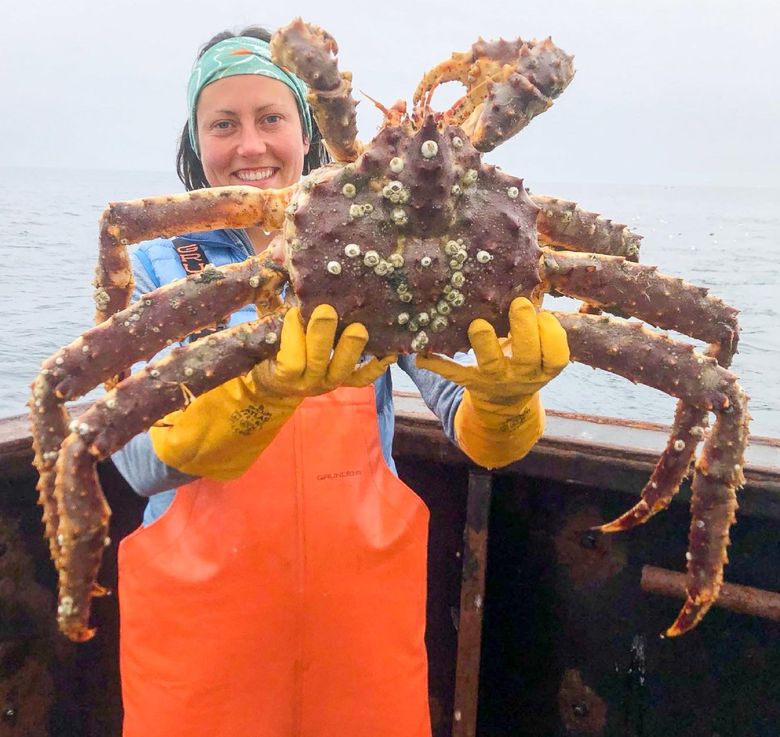In this striking photograph, a woman aboard a weathered, rusty crab fishing boat beams with pride as she presents an enormous king crab to the camera. Her teal bandana holds back her hair, while bright yellow latex gloves and vivid orange fisherman's coveralls protect her from the cold and wet conditions. The long-sleeved shirt peeking out from beneath her coveralls is a contrasting blue. The massive king crab, covered in barnacles, is held towards the viewer, displaying its gigantic, reddish-brown body and incredibly long legs—each leg appears longer than the woman's forearm. The background reveals the dark, weathered wood and metal sides of the boat's interior, with a glimpse of the ocean's surface and a foggy sky beyond. Her radiant smile and sparkling blue eyes capture the sheer joy and excitement of what is likely one of the largest crabs she has ever seen.